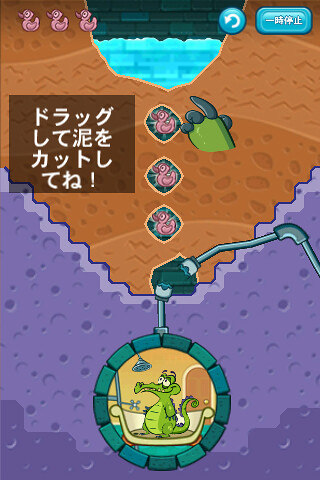This detailed screenshot from the mobile game "Where's My Water?" by Disney features a graphic scene requiring the player to draw a trail through dirt to guide water to a small green alligator named Swampy in a bathtub. At the top of the image, a half-filled pit of water is encased in dark blue and gray bricks and surrounded by brown sand-like dirt. On the upper left, three pink ducks icons are visible, and on the upper right, there are buttons: a circular arrow for a reset and a rectangle with Asian characters. 

In the middle section, a translucent gray rectangle with more Asian characters appears, and alongside this, there is a series of three diamonds showing graphics of the pink ducks, one in each diamond. Exiting from the brown dirt area is an alligator-like claw, seemingly belonging to Swampy. 

Further down, the image transitions to a blue section featuring a circular medallion bordered with greenish-blue tiles. Inside this circle, Swampy, a cartoon alligator, stands in a bathtub under a metal showerhead, showcasing the main objective of the game: guiding water to help Swampy complete his shower.